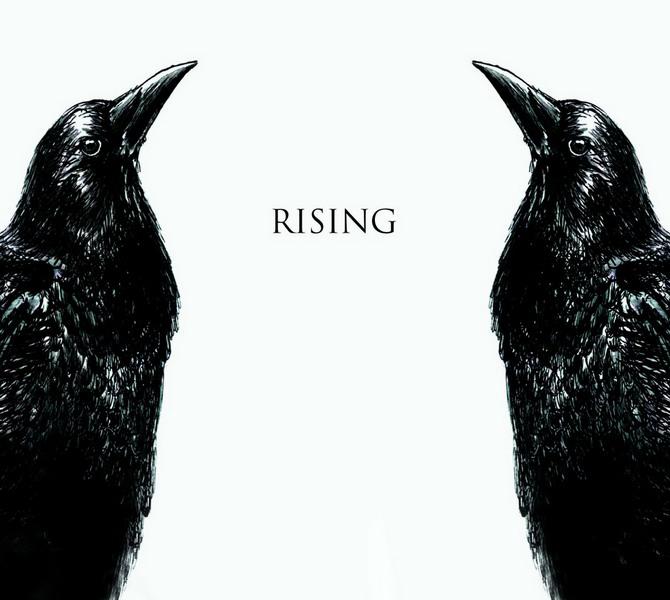The image features a medium light gray square background with the word "RISING" prominently displayed in all caps and black letters in the center. Flanking either side of the word are two black crows, which appear to be mirror images of each other. Each crow has a black beaded eye, a black sketched beak of medium length with a pointed end, and a black head adorned with white spots. The crows face each other from opposite sides of the image, with their beaks and bodies angled upwards, almost creating a bridge-like formation if they were closer together. Their backs are cut off by the edge of the frame, emphasizing their upward gaze and symmetrical positioning. There are no other details or text in the image beyond the crows and the word "RISING."